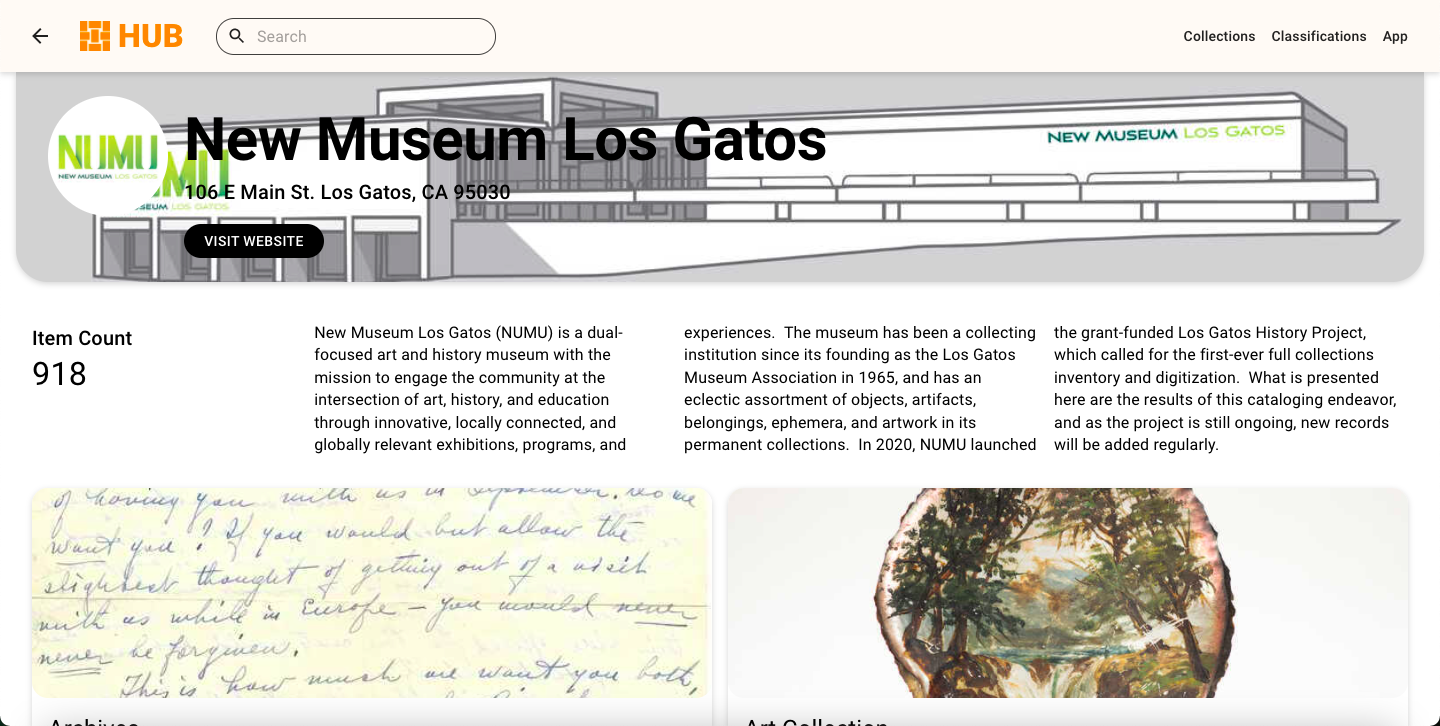The image appears to be a screenshot of a webpage showcasing the New Museum Los Gatos, located at 106 East Main Street, Los Gatos, California, 95030. The top banner features a back button on the left, followed by an orange woven symbol labeled 'Hub'. On the right side of the banner are menu options for 'Collections', 'Classifications', and 'App'. Below this is a thicker banner displaying a circular symbol with 'Numu', and text identifying the museum along with the address and a 'Visit Website' button. The banner is overlaid on a gray architectural drawing of the museum. Below this, the webpage shows an item count of 918 and three blocks of descriptive text detailing the museum's focus on art, history, and education. There is an emphasis on the museum's ongoing cataloging project, which regularly updates its collection of diverse objects, artifacts, and artwork, a practice rooted in its history since being founded as the Los Gatos Museum Association in 1965. The bottom third of the image features a handwritten note in blue and black ink, alongside a piece of artwork depicting a waterfall with overhanging trees.